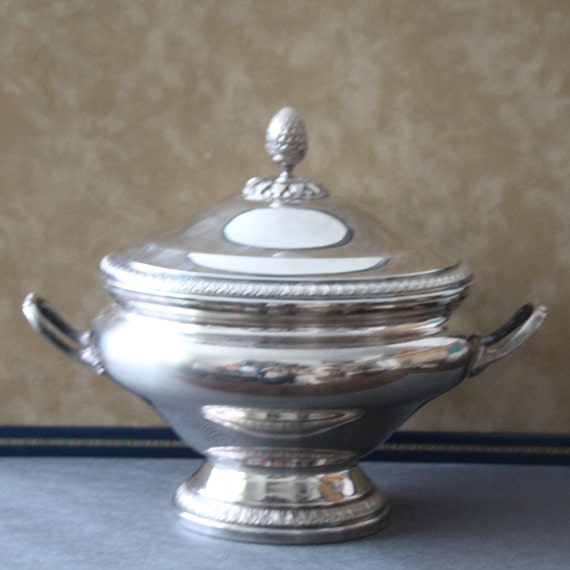In this square indoor photograph, an ornate silver container with handles on either side and a lid featuring a pineapple-shaped handle is prominently displayed. The container sits on a light blue surface, which could be a table, floor, or countertop. The background reveals a wall painted in a mix of tan and lighter cream blotches, with a thin stripe of dark navy blue adorned with a faint gold line running horizontally near the base. The silver surface of the container reflects light, highlighting its intricate patterns and designs, giving it an antique, royal appearance.